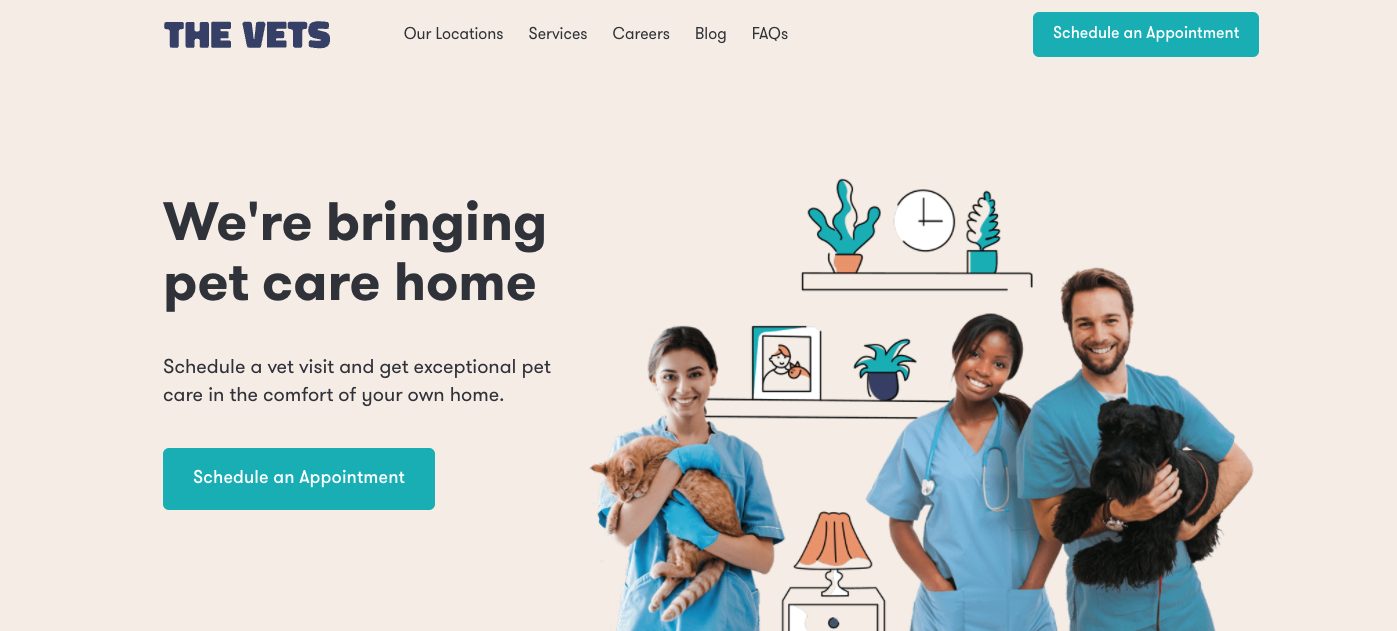The image showcases the homepage of the VETS website. In the upper left-hand corner, the word "VETS" is prominently displayed in all capital letters and blue coloring. To its right, near the top center of the page, is a horizontal menu bar with options including "Our Locations," "Services," "Careers," "Blog," and "FAQ." Further to the upper right-hand corner, there is a noticeable "Schedule an Appointment" button in an aqua greenish-blue hue with white text.

Central to the image, an eye-catching headline reads "We're Bringing Pet Care Home" in large font, positioned slightly to the left of center. Below this, a subheading encourages visitors to "Schedule a VET visit and get exceptional pet care in the comfort of your home." Beneath this text is another "Schedule an Appointment" button.

Dominating the lower section of the image, there are three veterinary professionals dressed in blue smocks. Two females and one male are featured, each holding a pet; one female has a cat, while the other female and the male are holding dogs.